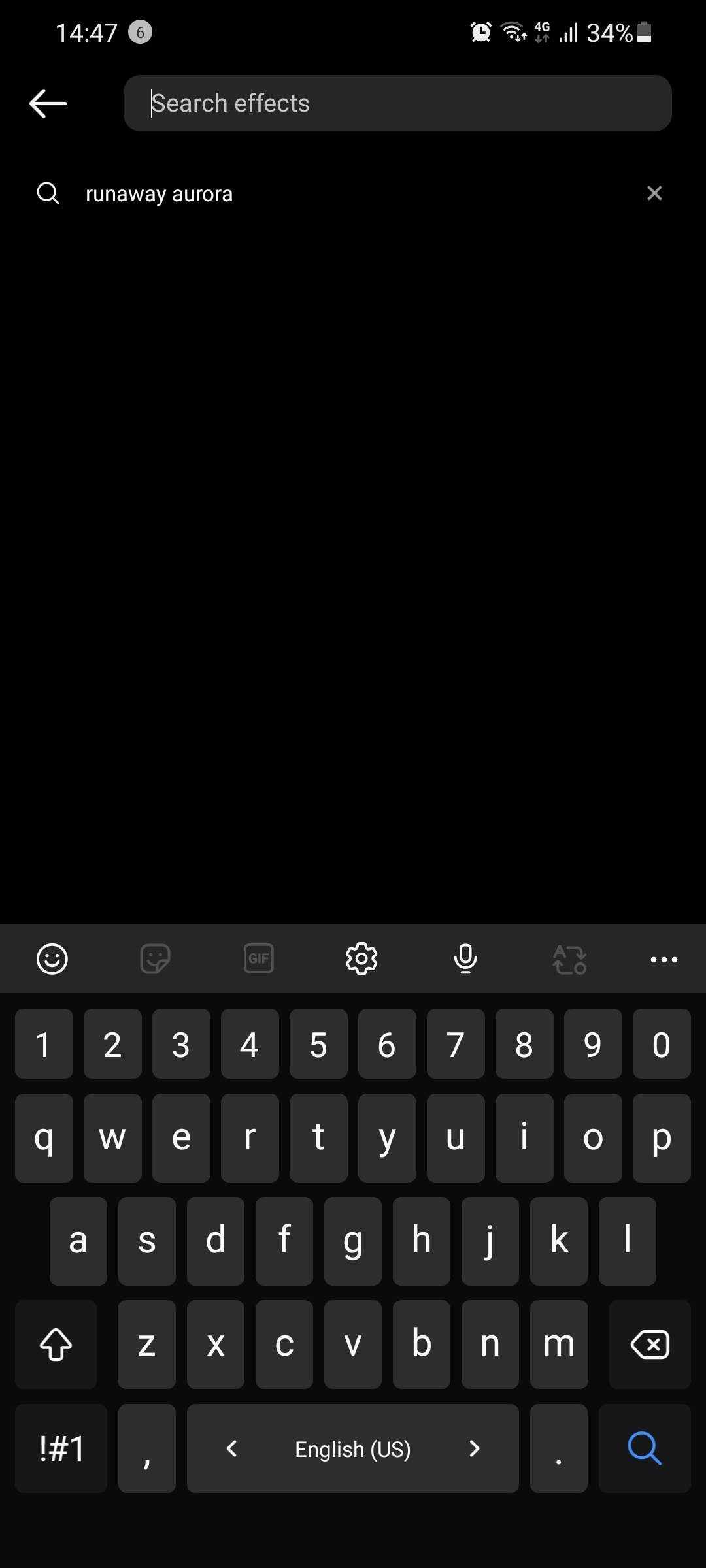The image is a screenshot of a digital search interface, likely from a smartphone or a similar device. At the top left corner, the time is displayed as 14:47 (2:37 PM). The top right corner features several icons in sequence: an alarm clock icon, a WiFi symbol, two signal bars labeled "4G," a mobile data indicator, and a battery icon showing 34% charge remaining. Below these status indicators, there is a grey search box with white text. Inside the search box, the placeholder text reads "Search effects." Beneath this, one of the previously searched terms is visible, "runaway aurora," also in white text. On the far right side of the search box, there is a small "X" icon, presumably to clear the search field.